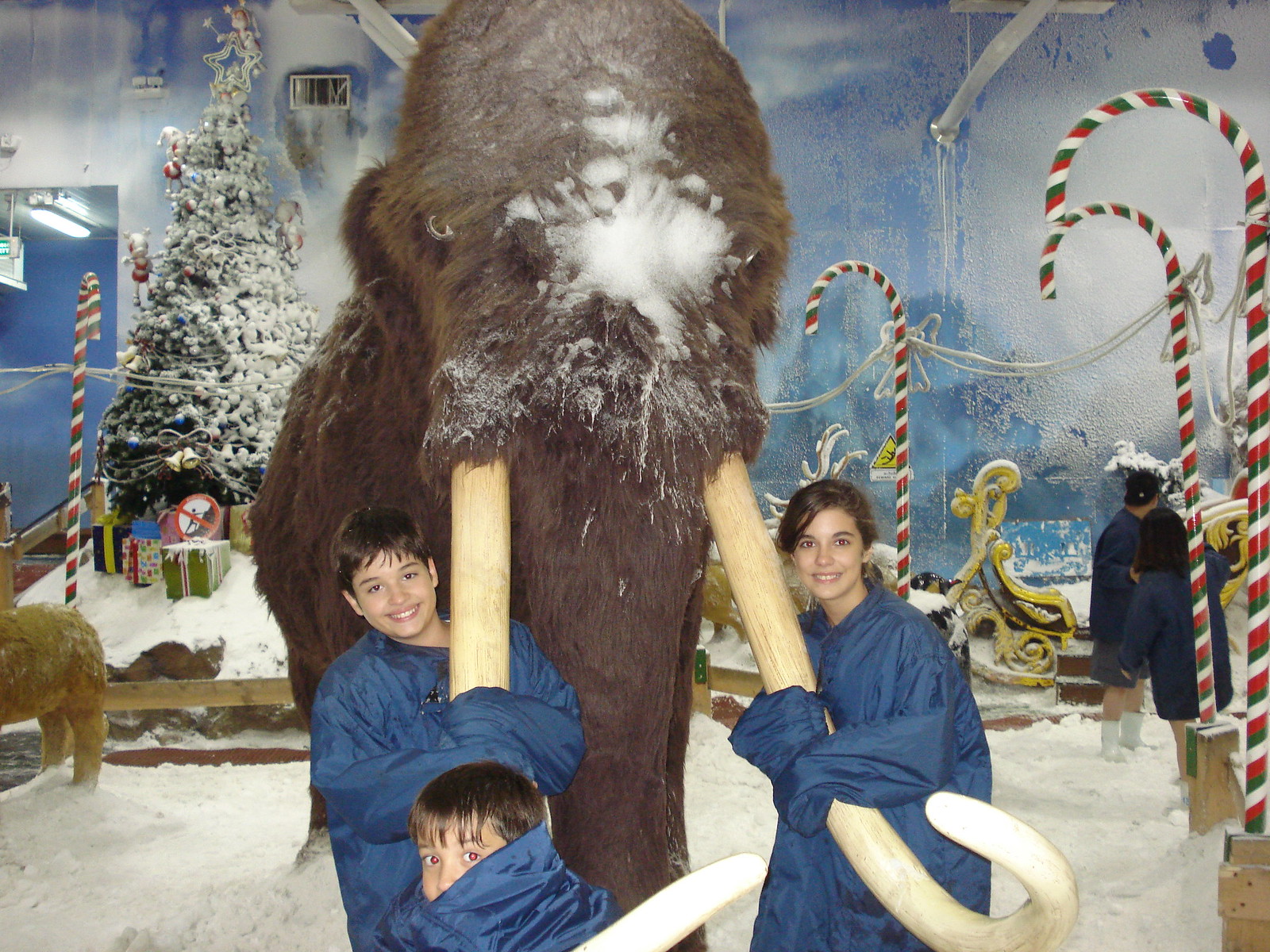In this Christmas-themed exhibit, set within what appears to be a museum, three children are joyfully posing with a life-sized model of a woolly mammoth at the center of the scene. The children, dressed in blue coats or snuggies, are warmly embracing the mammoth's enormous curved tusks, smiling brightly for the camera. The setting is rich with festive decor, including towering candy canes with green, red, and white stripes, which serve as decorative posts along the path. To the left, a Christmas tree dusted with fake snow stands proudly, surrounded by wrapped presents, enhancing the holiday spirit. The scene is further accentuated by a layer of fake snow covering the ground and the mammoth itself. The indoor environment, with light blue walls and white accent imitating snow, features an air vent above the Christmas tree and a doorway to its left. Additional people can be seen in the background, some next to what seems to be Santa's sleigh, adding to the bustling, touristy atmosphere of this winter wonderland exhibit.